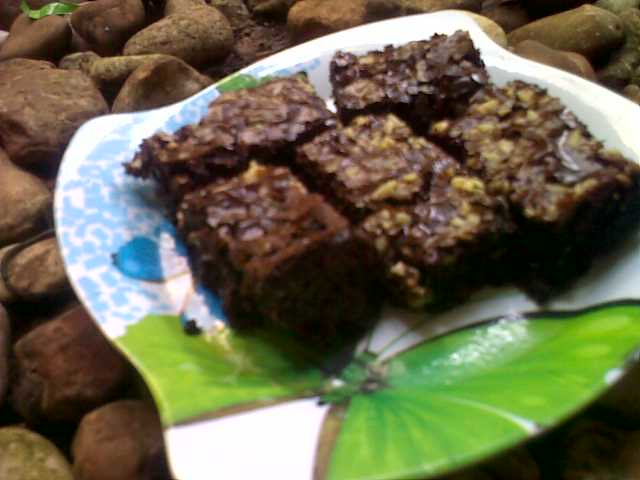This photograph captures a white ceramic or glass plate with a unique rounded square shape, adorned with vibrant designs including a prominent green butterfly and hints of blue patterns. The plate sits against a backdrop of large, reddish-brown rocks that provide a textured, natural setting. On the plate, there are five rectangular brownies, each dotted with yellowish-brown walnuts, their crispy tops suggesting they are freshly baked. The arrangement of brownies features three placed vertically in the front and two horizontally in the back. Notably, the brownie on the left-hand side seems to have a chunk missing, as if someone took a bite or a tear. The close-up focus on the brownies and the artistic plate highlights the intricate details of both the dessert and the backdrop, merging culinary and natural elements in one visually engaging image.